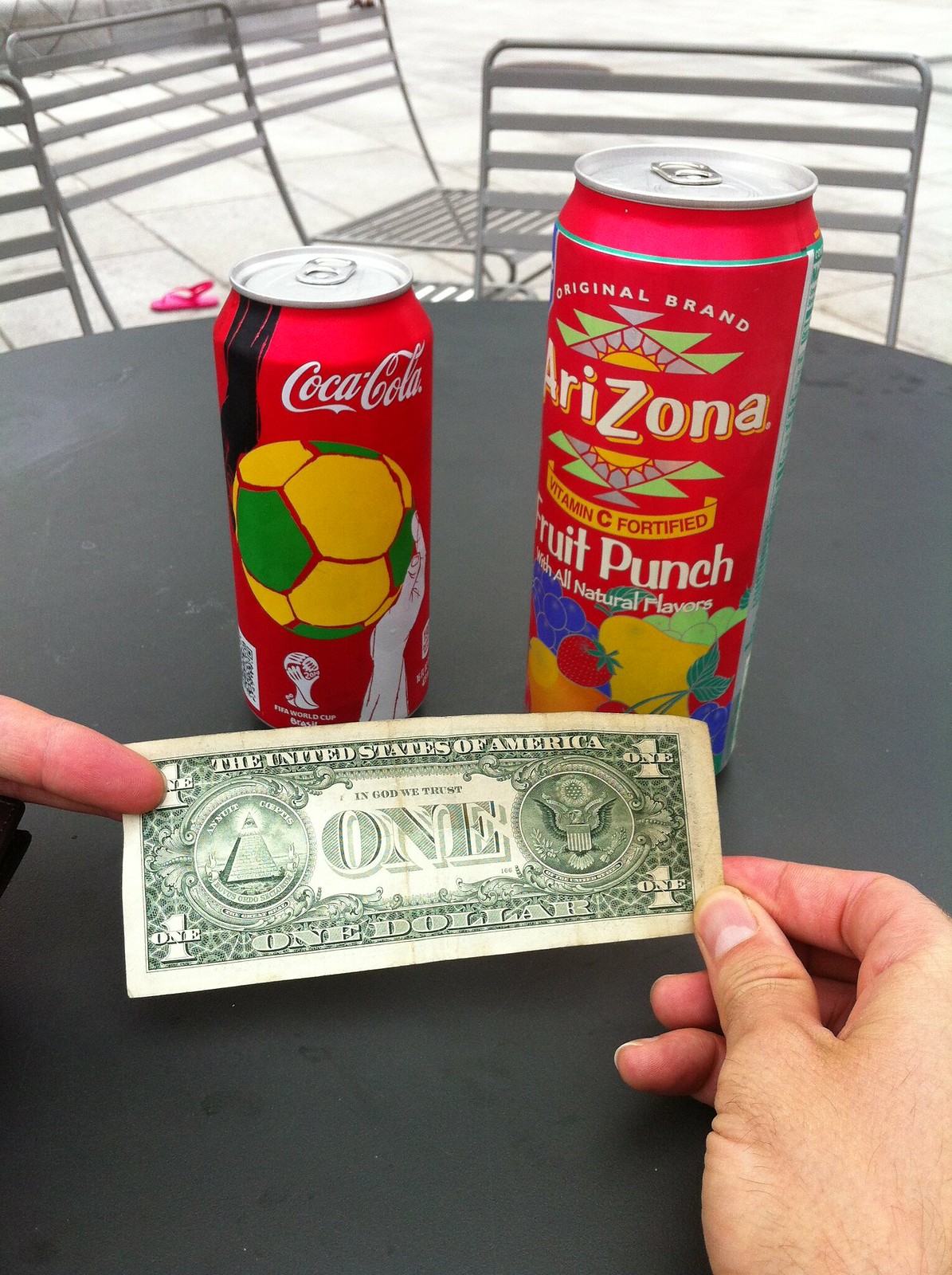This image captures a scene from a first-person perspective, as if taken from the viewpoint of someone seated at a dark gray table outdoors on a white stone patio. Three metal chairs can be seen positioned behind the table. In the center of the table, two white hands, appearing to be Caucasian with a bit of hair, are holding up the back of a U.S. one-dollar bill. On the left side of the table is a red Coca-Cola bottle with its iconic white text, while on the right side is a red can of Arizona Original Brand Iced Tea Fruit Punch, clearly labeled as fortified with Vitamin C and featuring all-natural flavors. Additionally, there's a distinctive yellow soccer ball with green details visible on the left side of the scene.